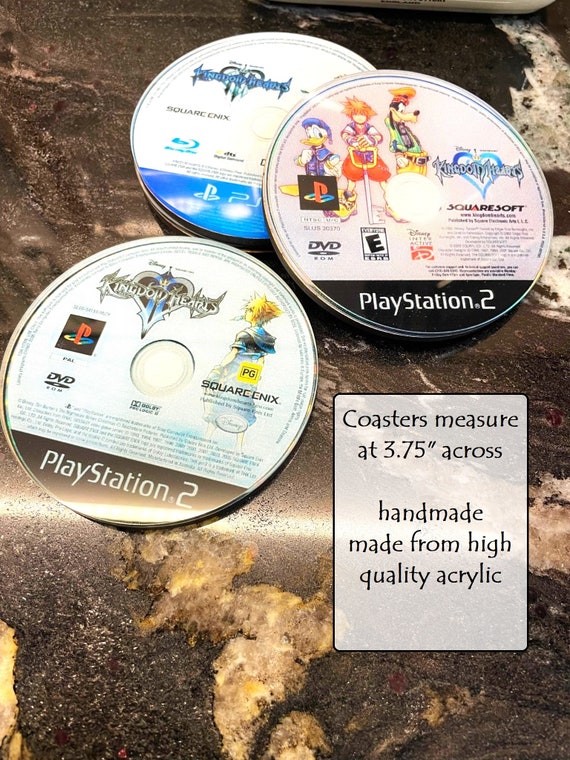This image appears to be from an eBay-style advertisement listing for handmade coasters designed to look like PlayStation 2 game discs. The three coasters, meticulously crafted from high-quality acrylic, each measure 3.75 inches across. The coasters mimic the appearance of the discs for the popular Kingdom Hearts series, including Kingdom Hearts, Kingdom Hearts 2, and Kingdom Hearts 3, with vivid designs featuring anime and Disney characters. They are arranged on a striking granite countertop, characterized by its black stone interspersed with white flecks and intricate geodesigns. A sign in the bottom right corner details the dimensions and materials of these unique items, highlighting their artisanal quality.